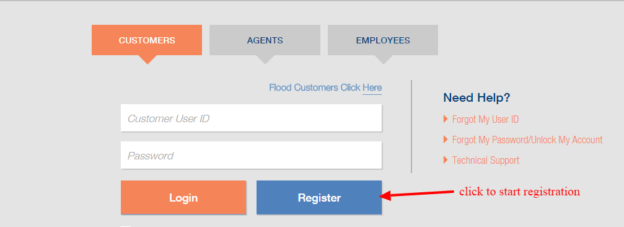The image displays a login screen for a website, featuring a sleek and organized design. At the top of the screen are three tabs labeled "Customers," "Agents," and "Employees." These tabs are grey with blue text, while the selected tab is highlighted in orange with white text.

The entire page has a light grey background. Below the tabs is a blue link that reads "Flood Customers Click Here." The main section of the login interface consists of two input fields for "Customer User ID" and "Password." Beneath these fields, there is an orange "Login" button and a blue "Register" button.

On the right side of the screen, a sidebar header titled "Need Help?" offers assistance. This sidebar includes four orange links: "Forgot My User ID," "Forgot My Password," "Unlock My Account," and "Technical Support." At the bottom of this sidebar, there is a message that says "Click to Start Registration," accompanied by a red arrow pointing towards the "Register" button.